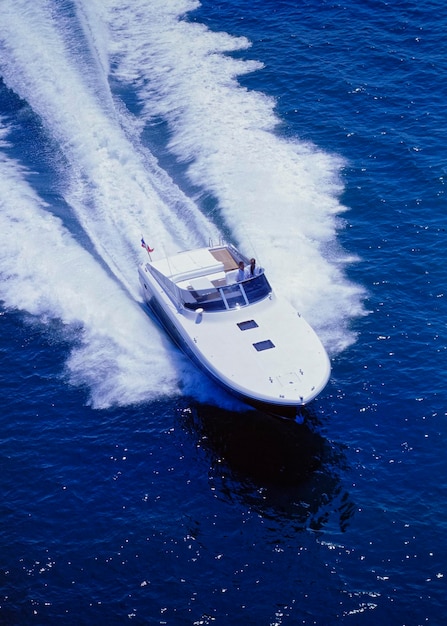This is a detailed portrait-oriented photograph taken from above, depicting a white speedboat slicing through the dark blue ocean on a sunny day. The speedboat, heading from the top left towards the bottom right of the frame, creates a striking visual with three distinct streams of white wake trailing behind it, indicating its high speed. The water around and behind the speedboat is a stunning deep blue, with light reflections adding a dynamic sheen to the scene. The boat features two dark rectangular porthole windows at the front and a three-section windshield. Two people, both dressed in white shirts, are visible at the steering wheel. Additionally, a flag flutters from the back left side of the boat, further enhancing the lively maritime atmosphere of the image.